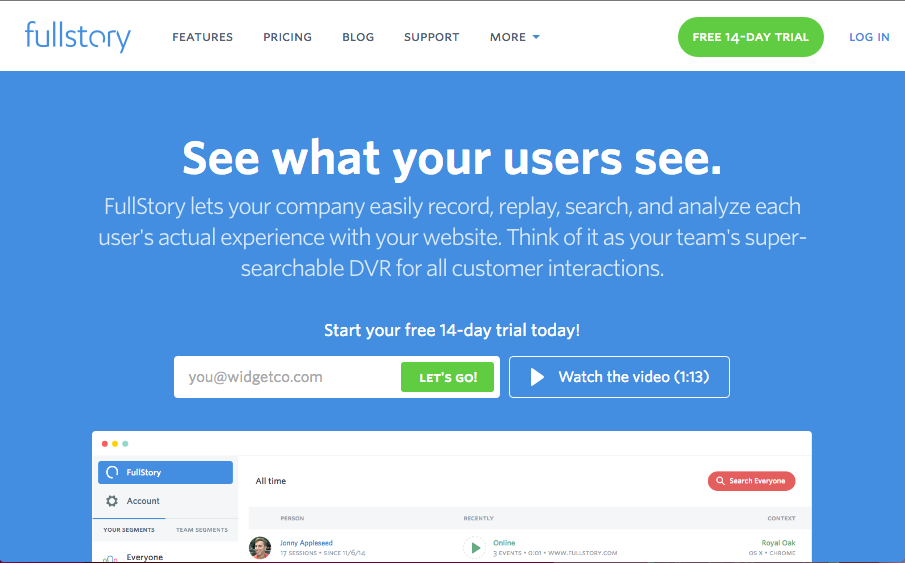The image depicts the homepage of FullStory's website, a company specializing in user experience analytics. In the top left corner, the company logo, "FullStory," is displayed in blue. To the right of the logo, a navigation menu features the options: Features, Pricing, Blogs, Support, More, alongside a prominent call-to-action button labeled "Free 14-Day Trial" in white text on a green background. A blue hyperlink offers the option to log in.

Centered on the page, a bold headline in white text declares, "See what your users see." Accompanied by a concise description, it explains FullStory's service, emphasizing its capability to record, replay, search, and analyze every user's interaction with your website. The text describes the tool as a "super searchable DVR for all customer interactions," providing a clear value proposition against a solid blue background.

Midway down the page, another call-to-action button invites users to "Start Your Free 14-Day Trial Today," flanked by an input box for entering an email address. Adjacent to this, a clickable element allows users to watch an explainer video. Just below, the webpage prominently features a video box, giving a preview of the FullStory service in action. The layout and design effectively guide the viewer’s attention through the key offerings and actions available on the homepage.